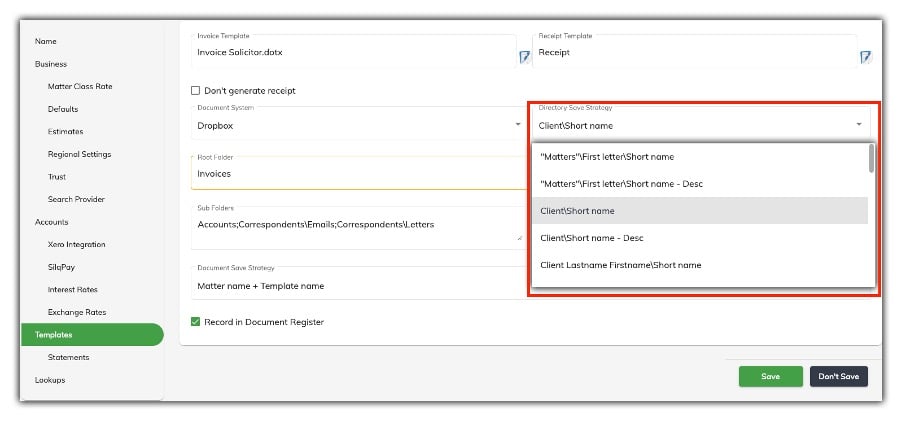This is a detailed screenshot of the settings menu in an application or website, presented as a long vertical rectangle. On the left side, there's a gray column with black vertical text listing various menu options. From top to bottom, the options read: "Name," "Businesses," "Master Class Rate," "Defaults," "Estimates," "Regional Settings," "Trust," "Search Provider," "Accounts," "Zero Integration," "Silk Pay," "Interest Rates," "Exchange Rates," "Templates," "Statements," and "Lookups." The "Templates" option is highlighted with a green oval, indicating it is currently selected.

On the right side of the screenshot, a white panel corresponding to the "Templates" selection is visible. This panel displays further options at the top, labeled "Invoice Template" and "Receipt Template." Under "Invoice Template," there is a file name, "invoice_solicitor...x," partly visible.

In the lower right corner, there are two action buttons. One is green and labeled "Save," while the other is black and labeled "Don't Save," both with white text.